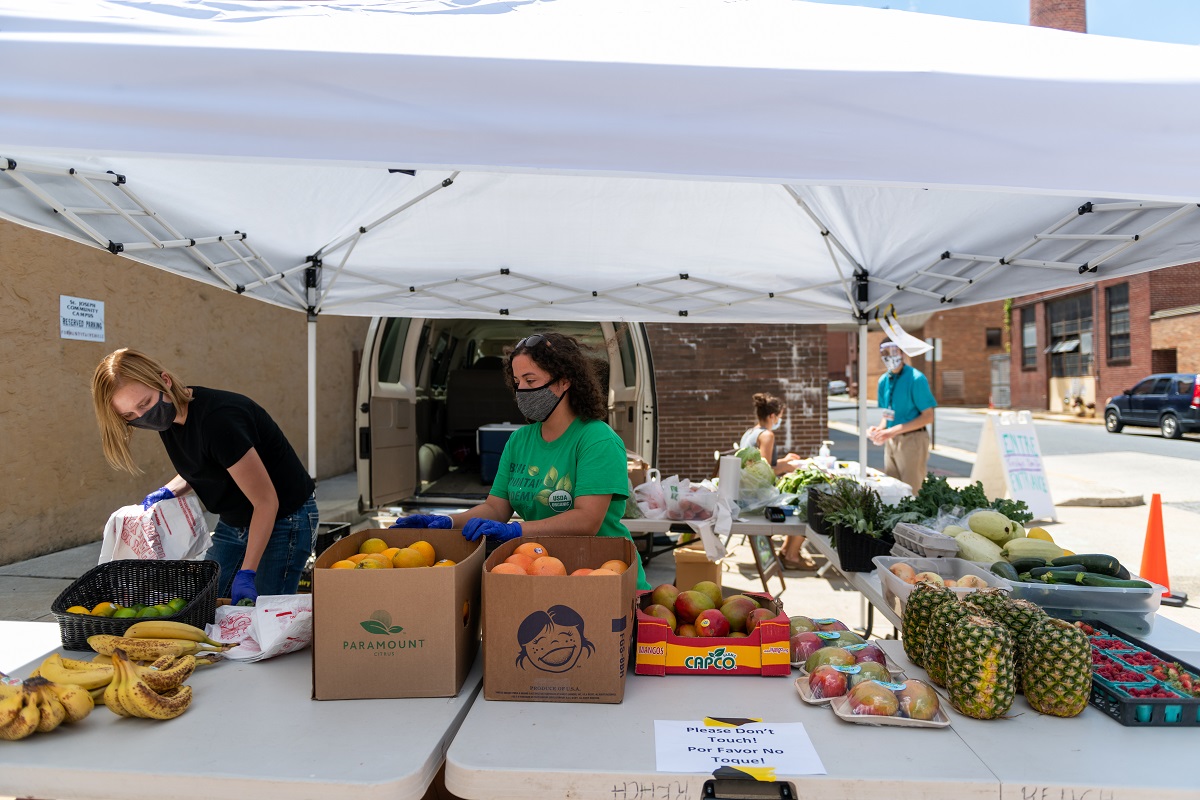In a bustling corner of a town with red brick buildings lining the streets, a vibrant farmer's market is set up under a pop-up white canopy tent. The tent shelters a U-shaped arrangement of six white tables, groaning under the weight of a colorful bounty of fruit and vegetables. Bananas, peaches, mangoes, pineapples, citrus fruits, apples, bologna, and cartons of eggs are among the diverse produce, alongside vegetables like zucchini. Three workers, all wearing black face masks and blue gloves, are busily arranging the items on the tables. One woman, wearing a green shirt, appears to be overseeing the operation. In the background, another woman is seated at a table, possibly handling money or recording transactions. A parked, open van sits beneath the tent, indicative of recent or ongoing deliveries. The surrounding area features a street on one side, a warehouse, and on the other side, a somewhat boarded-up area. This scene depicts a lively yet cautious community activity, suggestive of a period during or following the COVID-19 pandemic.